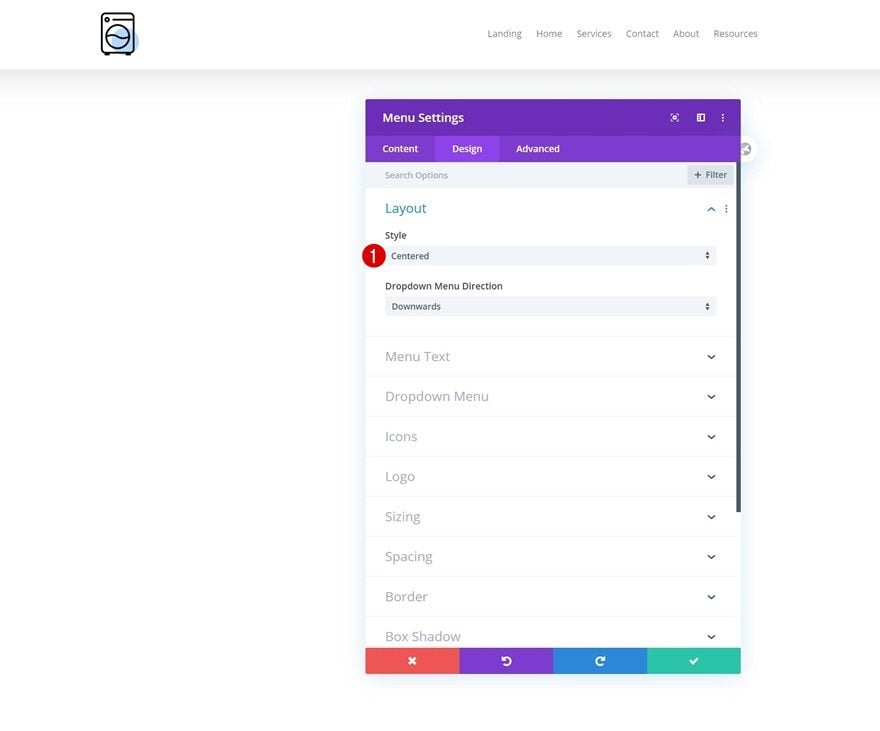The image depicts a detailed screenshot of a web page or application interface. On the left side, there is a graphic of a black front-loading washing machine, partially filled with water. The right side features a navigation menu with the options: "Landing," "Home," "Services," "Contact," "About," and "Resources," all presented on a clean white background.

A vertical, rectangular pop-up screen is prominently displayed, featuring a purple banner at the top. On this banner, the text "Menu Settings" is displayed in white. To the right of this text are an expand button and three additional buttons. The banner has three tabs labeled "Content," "Design," and "Advanced," with the "Design" tab currently active, highlighted by a lighter shade of purple.

Below the banner, there is a search bar and a filter button marked with a plus symbol. The section includes various layout options, indicated by blue text and an upward-pointing arrow. The category "Style" is highlighted, with an adjacent red circle enclosing the number one. A dropdown menu positioned downward lists available styles, with the current selection being "Centered."

Additional menu options include "Menu Text," "Drop-down Menu," "Icons," "Logo," "Sizing," "Spacing," "Border," and "Box Shadow," each presumably offering further customization settings for the interface design.